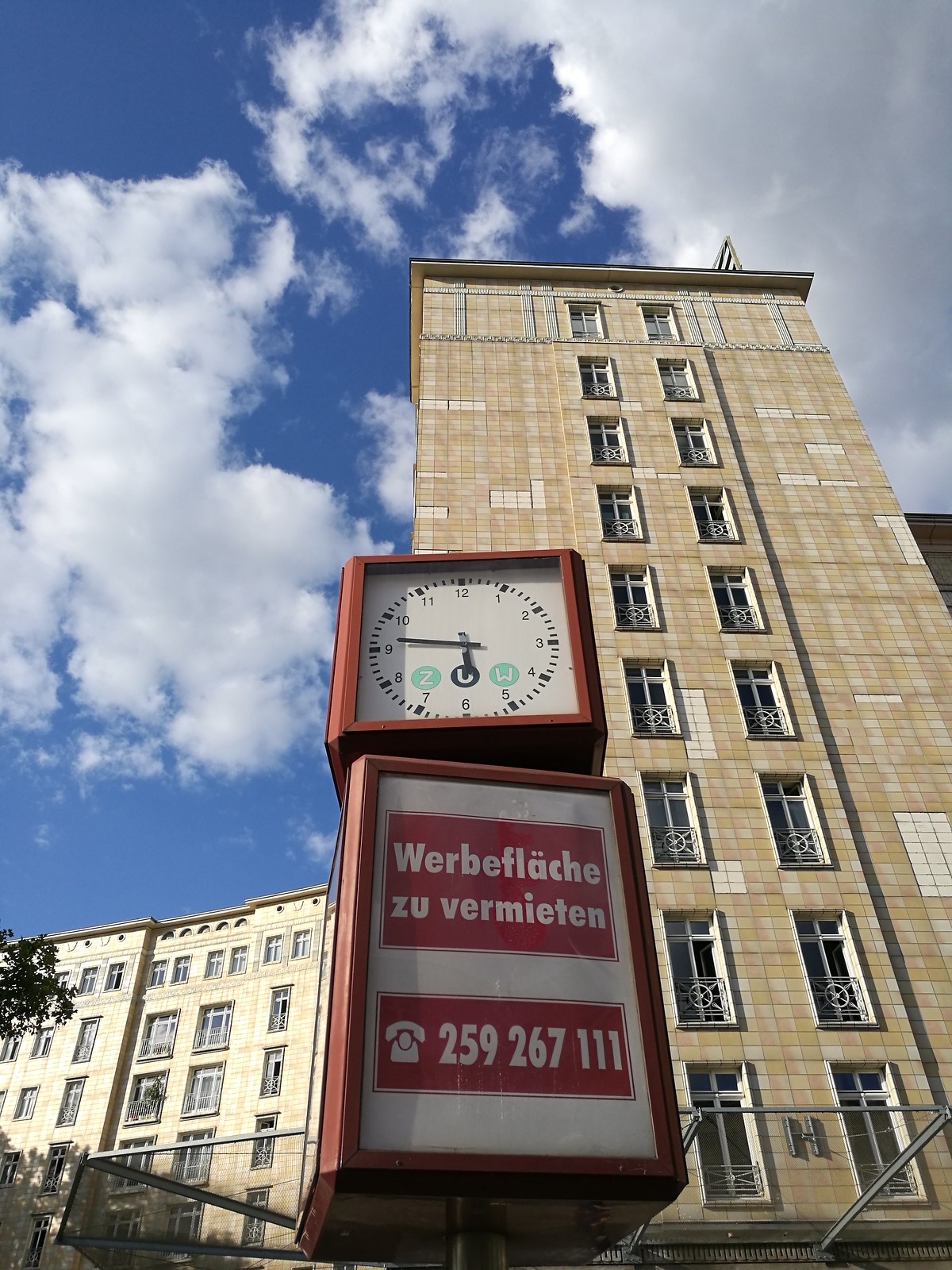The image showcases a tall, yellow building adorned with multiple windows arranged in two vertical rows extending from the top to the bottom. Each window features a circular design element and a railing. The building's façade is comprised of numerous square tiles, giving it a distinctive and structured appearance. Above the entrance, there is a rectangular white sign outlined in red, displaying a phone number and some text. Positioned above this sign is a clock, also outlined in red, with a white face, black hands, and two bluish-green circles on it. The sky in the background is a clear blue interspersed with a few white clouds, adding a serene backdrop to the scene. To the left of the main building, another yellow building with numerous windows is visible, enhancing the urban setting of the picture.